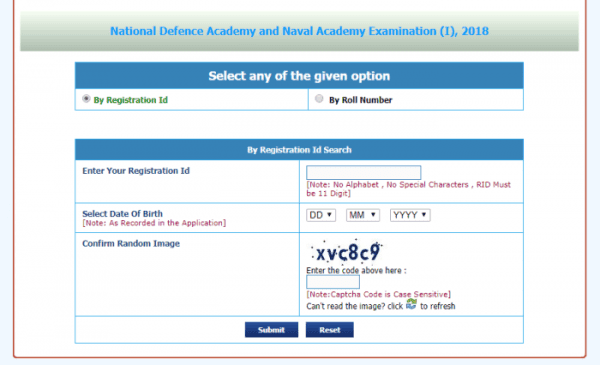**Detailed Description of National Defense Academy and Naval Academy Examination 2018 Registration Page:**

The image depicts a registration form for the National Defense Academy and Naval Academy Examination (I), 2018. The form is designed with a predominantly blue and white color scheme. 

At the top, there is a blue box with white lettering that reads: "Select any of the given options." Below this, the options are listed from left to right: "By Registration ID" (highlighted in green to indicate its selection) and "By Roll Number."

Moving further down, there is a blue banner with white letters that says: "By Registration ID Search."

The form then prompts the user to: 
1. "Enter your registration ID"
2. "Select date of birth" (noted as recorded in the application)
3. "Confirm random image."

To the right, there is an empty text box with the following red warning note below it: "Note: No alphabet, no special characters, our ID must be 11 digits."

For the date of birth, the form provides selections for date, month, and year. Additionally, there is a displayed CAPTCHA code: "XVC8C9," with instructions underneath: "Enter the code above here." An empty text box below this is meant for the CAPTCHA entry, with a red note beneath emphasizing, "Note: CAPTCHA code is case sensitive."

There is also a refresh option for the CAPTCHA beside the text: "Can't read image? Click to refresh." 

Towards the bottom of the form, there are two functional buttons, both blue with white lettering. One reads "Submit" and the other "Reset."

This detailed layout ensures proper user guidance through the registration process with clear visual and textual instructions.